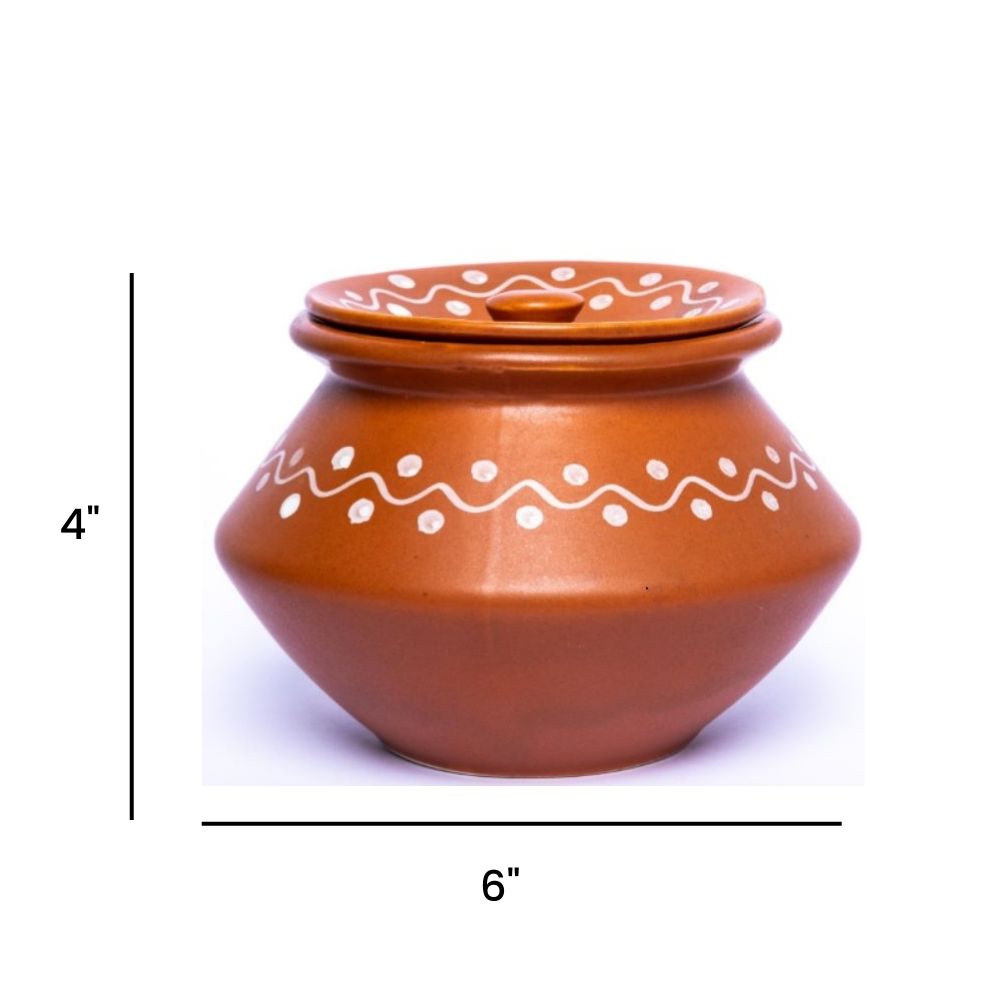This detailed image shows a close-up of a small terracotta ceramic container with a lid. The prominent color is brown, and it features a decorative design consisting of a white wavy line encircling the container, with small white dots positioned in the valleys created by these wavy lines. This pattern continues onto the lid. The container has a distinctive shape: it starts with a narrower base and widens towards its center, which is the widest part at six inches in diameter, before narrowing again towards the top. The height of the container is denoted by a black vertical line measuring four inches. The lid, which fits snugly into the lip of the container, has a plate-like appearance with a small knob at the center for easy handling. The image effectively displays both the artistic and functional aspects of this beautiful piece of pottery.